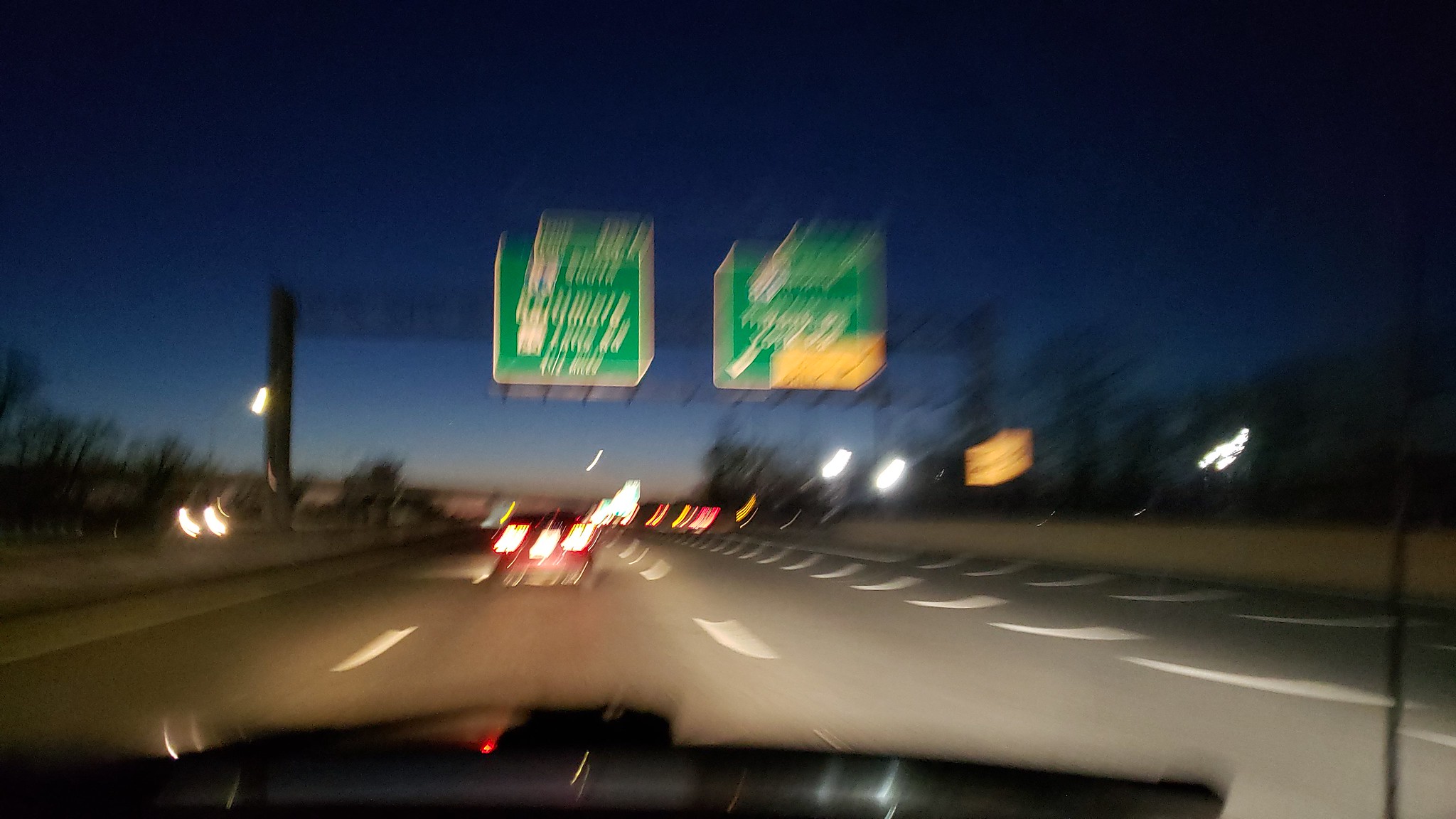This horizontal nighttime photograph portrays a blurred view from inside a moving vehicle, looking out through the windshield onto a three-lane interstate highway. The vehicle's black dashboard is partially visible at the bottom edge of the image. In the distance, ahead of the viewer, there is a red car with illuminated brake lights suggesting a recent deceleration. The scene is bathed in artificial light from streetlights and the bright headlights of an approaching vehicle on the opposite side of the median, which is divided by a short gray wall. 

Above the highway, two large green interstate signs loom, though the text on them is unreadable due to the motion blur. A yellow traffic sign is faintly visible behind the gray median to the right, possibly indicating an upcoming exit or caution. Meanwhile, the night sky dominates the background, with a faint sliver of the moon peeking out beside a pole to the left. The horizon appears slightly lighter, likely reflecting urban light pollution or the approaching dawn. Overall, the image captures the essence and busyness of a nighttime drive on a blurred, bustling interstate.